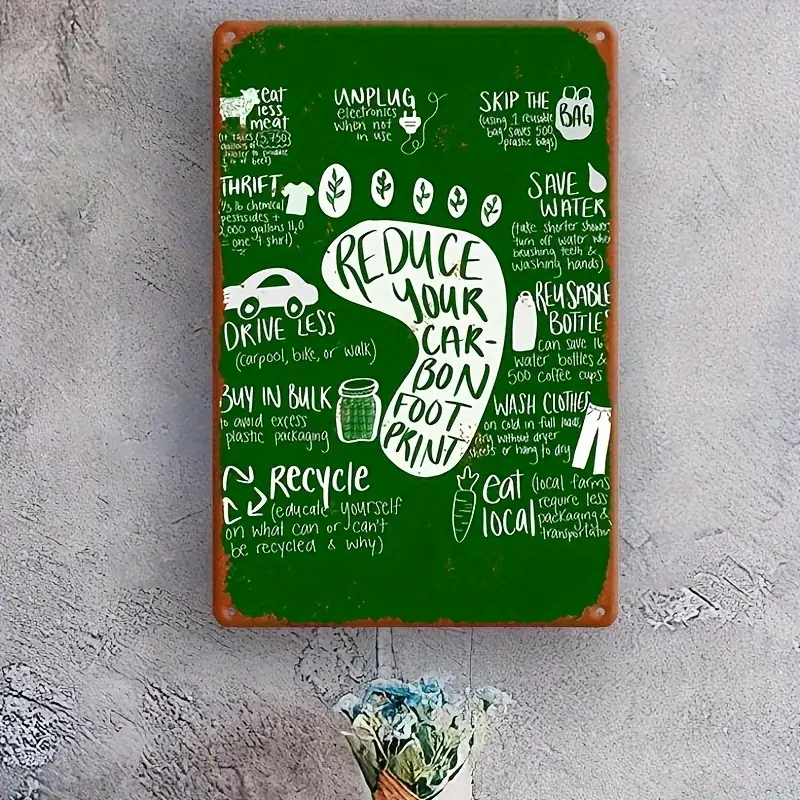In the image, we see a brown block with green parts that are fading, placed on a grey-colored platform. The background appears to be a grayish colored wall. The block features a central illustration of a foot with green leaves on the toes, which are not attached to the foot. The footprint includes the message "Reduce your carbon footprint," written in white text.

Around the footprint, there are several pieces of text and illustrations in white, each promoting eco-friendly actions. They include:

- "Eat less meat," accompanied by an image of a cow.
- "Unplug electronics when not in use," with a plug illustration.
- "Skip the bag," next to a white bag icon.
- "Thrift," illustrated with a t-shirt.
- "Drive less (carpool, bike or walk)," with a car icon.
- "Save water," next to a water drop.
- "Reusable bottle," illustrated with a bottle.
- "Wash clothes on cold and full loads," with a pair of jeans and a hanger drawing.
- "Eat local," accompanied by a carrot illustration.
- "Recycle," with the recycling symbol.
- "Buy in bulk to avoid excess plastic packaging," next to a salt shaker.

Illustrations next to these texts help to visualize each activity. Below this block, there is a bouquet of flowers, adding a decorative touch to the scene.